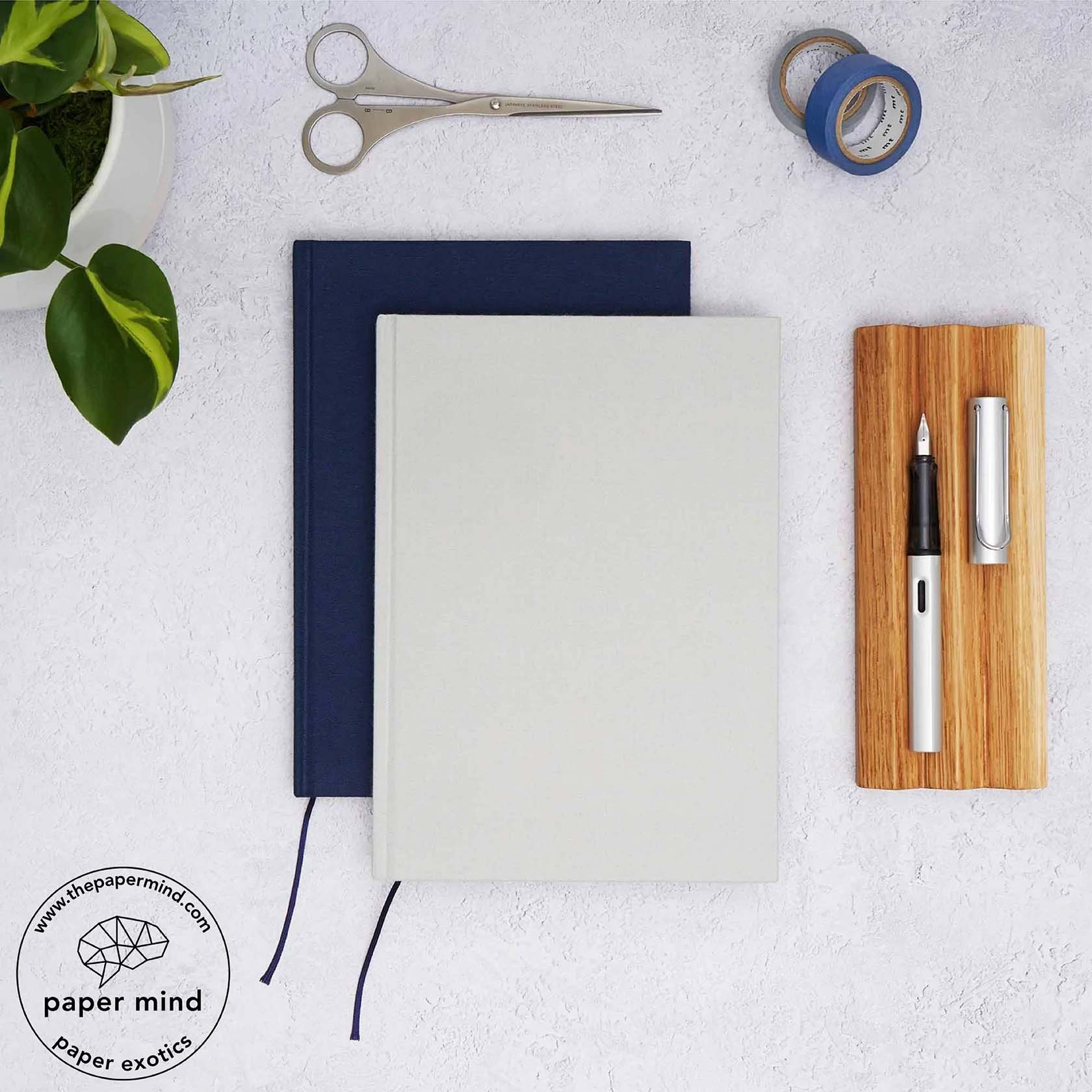The image is an advertisement for Paper Mind, showcasing their Paper Exotics collection with a logo and website, www.thepapermind.com, prominently displayed. At the center of the composition, placed on a white textured table, are two journals: an upper plain white journal and a lower navy blue journal, both featuring small sewn-in silk bookmarks peeking out. To the top-left corner of the image, a green plant in a white pot partially enters the frame. In the top-middle section sits a pair of silver scissors, while to their right, there are two rolls of tape—one blue, the other gray. On the right side of the journals, there's an old-fashioned pen resting on a wooden holder. The overall background has a marbled or clay-like appearance, adding a refined touch to the setup.